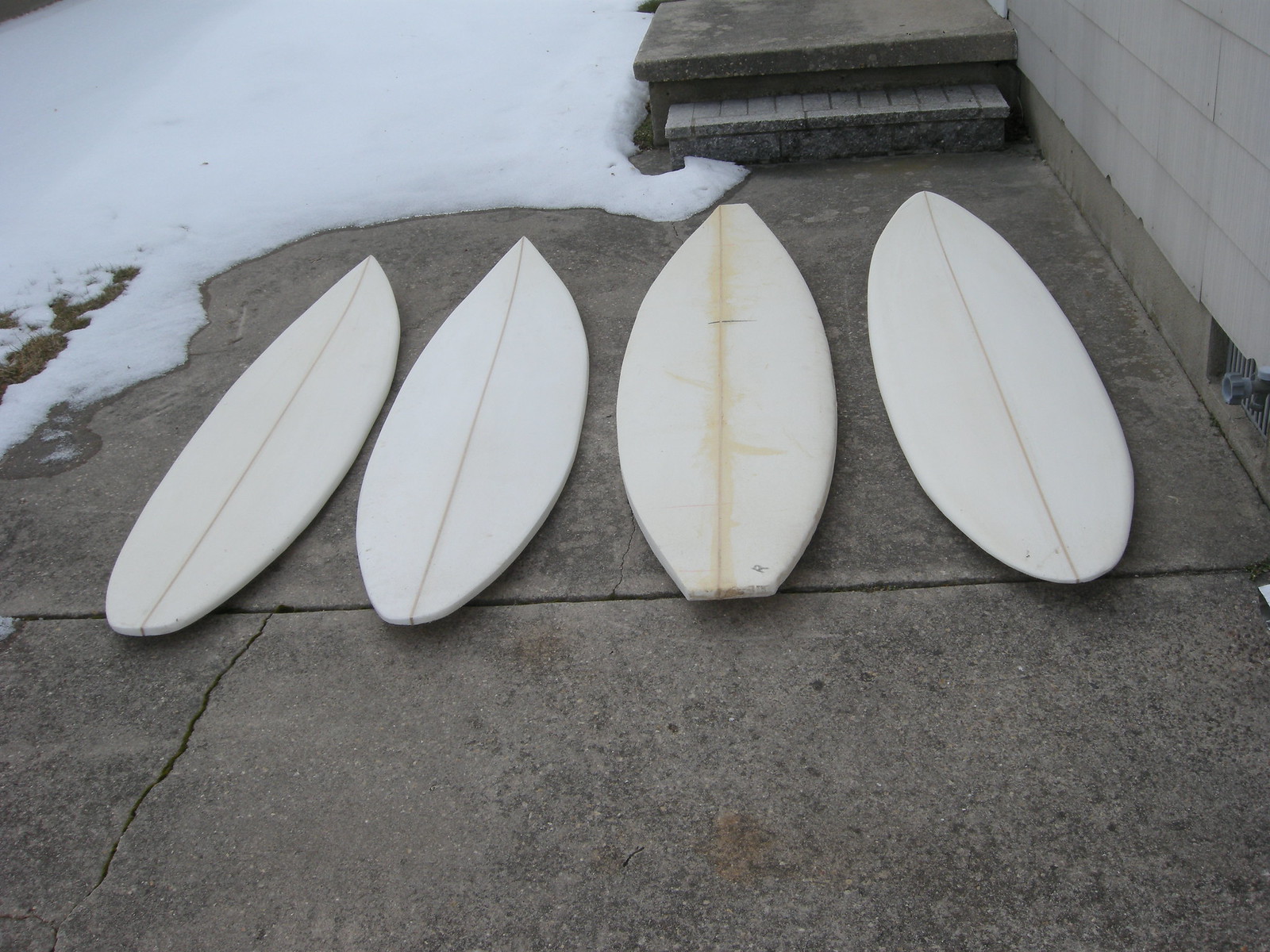This detailed photograph captures a wintry scene set against a backdrop of a white stone wall and concrete steps, one of which reveals visible bricks. In the upper left corner, a patch of melting snow exposes a segment of dark brownish-gray grass amid solid white snow. At the center, the slightly cracked, textured concrete pavement, predominantly gray with occasional black and orange spots, serves as the stage for four almost identical white surfboards. The surfboards, reminiscent of the color of white seashells with an off-white ivory hue, each feature a thin line down the center. Notably, the third surfboard from the left has a more diffuse, brownish line. The two surfboards on the left are slightly shorter than the others. The second surfboard from the right appears to have both ends snapped off, presenting a flat appearance, while the others maintain a rounded front end and a pointed back end. The incongruity of the surfboards against the snowy setting highlights their unexpected presence, as they rest aligned on the cracked concrete surface of what seems to be a house's sidewalk or driveway.